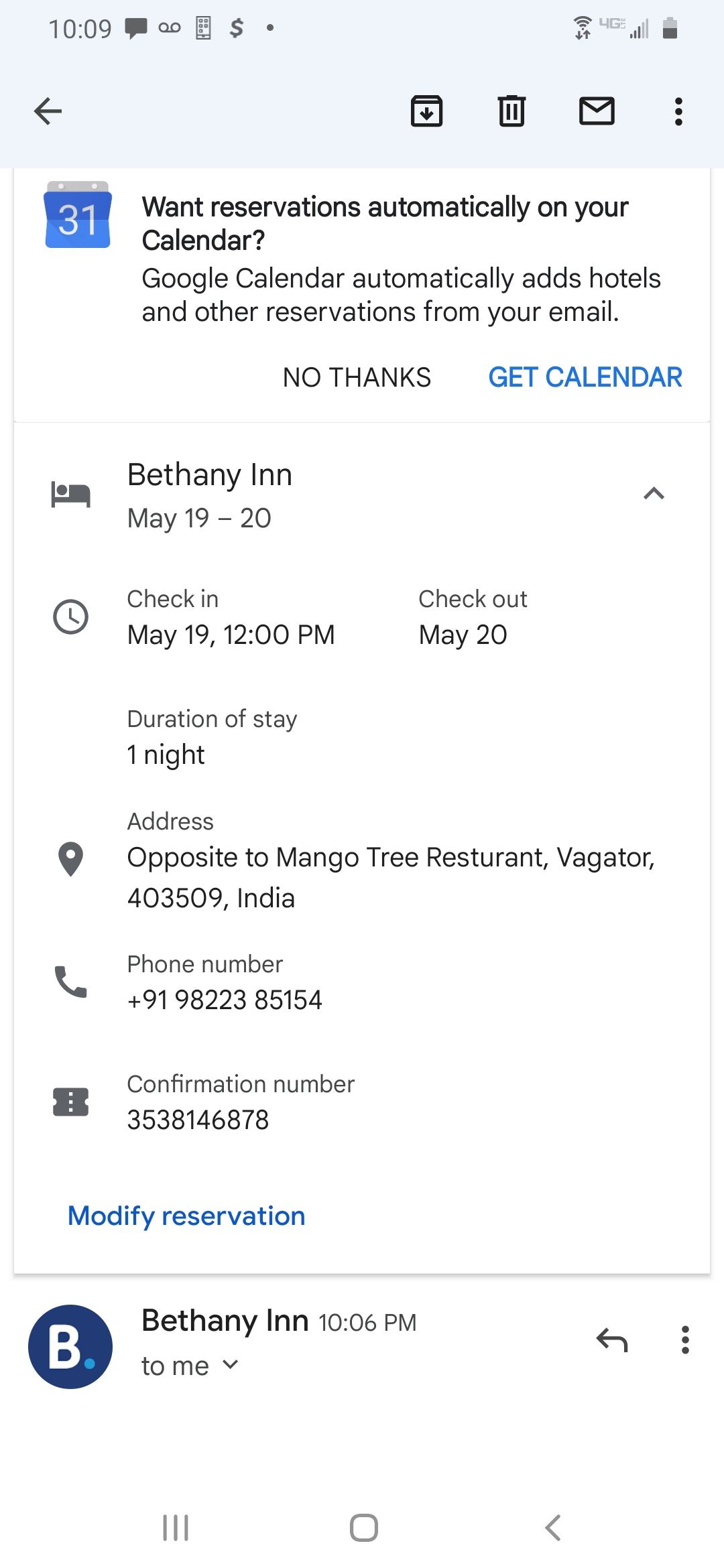A detailed screenshot captured from a smartphone at 10:09 with approximately 50% battery life shows a reservation for Bethany Inn. At the top, an informational banner prompts the user with, "Want reservations automatically on your calendar? Google Calendar automatically adds hotels and other reservations from your email," followed by options, "No Thanks" in black and "Get Calendar" in blue. Below the banner, a section with a bed icon is labeled "Bethany Inn, May 19-20." 

The next segment features a clock icon with details: "Check In, May 19, 12 PM. Check Out, May 20. Duration of stay, one night." Immediately below is an address section marked with a map pin icon: "Opposite to Mango Tree Restaurant, Vagator, 403-509, INDIA." The subsequent line, denoted by a phone icon, provides a contact number: "+91 9822385154." Following this, a ticket icon indicates the confirmation number: "3538146878." 

Toward the bottom, a blue link allows for "Modify Reservation." The content culminates with a dark blue circle featuring a white capital "B" and a small blue dot. Adjacent to this, it reads "Bethany Inn, 10:06 PM," above a blank message space.

This organized reservation information ensures a structured and detailed overview, making it easy for the user to verify the booking details and make any needed modifications.